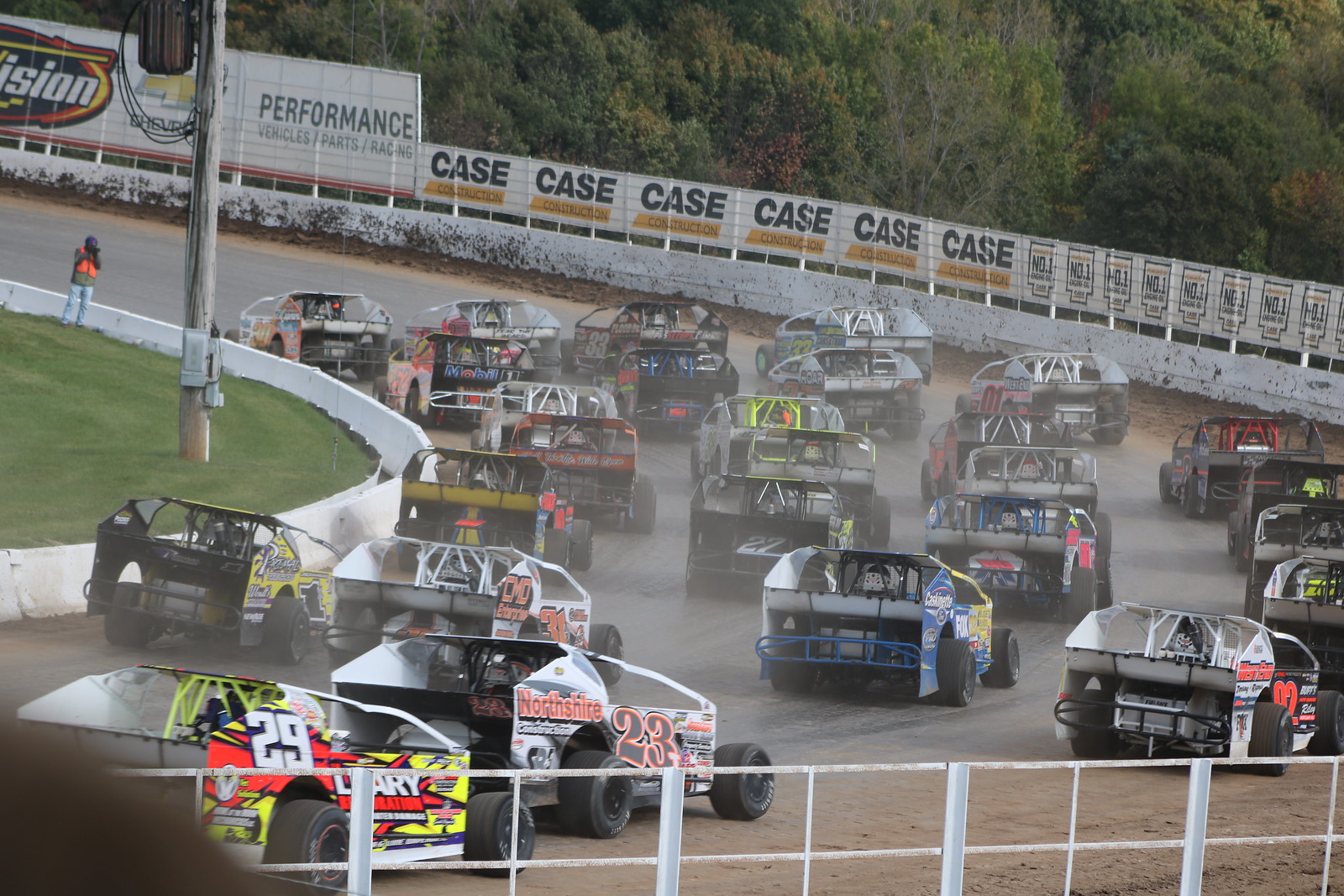The image captures a dynamic scene at a racetrack, focusing on a busy corner where approximately 15 to 20 small race cars, resembling a mix between go-karts and race cars, are maneuvering around the bend. The lower portion of the image features a small white barricade stretching horizontally from left to right, separating a strip of dirt from the track itself. In the middle and right sections, several cars are seen veering off into the dirt slightly, adding to the chaotic energy. 

To the left, another white fence outlines a grassy area with a pole and a person standing behind it, providing a sense of scale and human presence. The track disappears off the top left of the image, where a taller wall adorned with numerous advertisements, including a prominent one with the word "CASE" and another mentioning "performance vehicles, parts, and racing," runs parallel. Additionally, a larger sign mentions "Chevrolet" and "performance" partially peeks into the frame from the upper left. 

In the background, lush trees frame the upper right corner, contrasting the mechanical scene with nature. A hint of smoke and various colored decals on the cars, each adorned with different numbers and sponsors, underscore the intensity of the race. Flags bearing the name "CASE" dot the sidelines, reinforcing the sponsorship presence, while a safety person stands vigilantly nearby, ensuring the proceedings go smoothly.